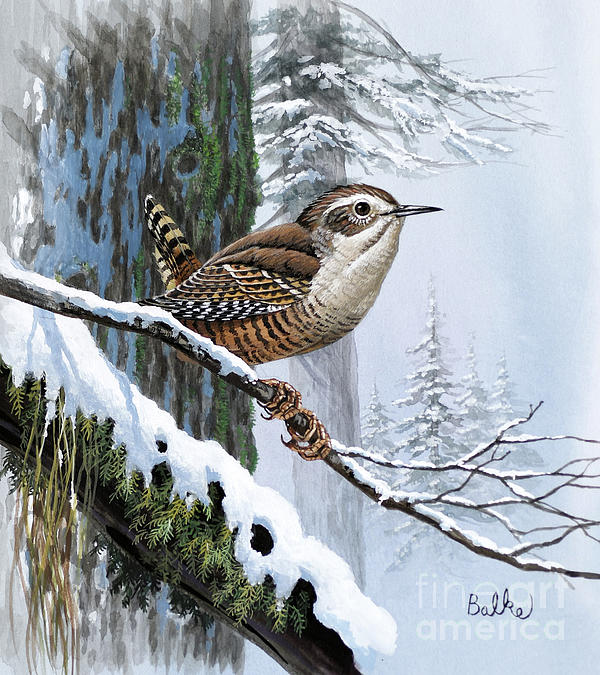In this detailed painting, a bird resembling a sparrow perches on a slender, snow-covered branch. The bird is depicted in a side view, allowing a clear view of its brown, patterned feathers and small, sharp black beak. This branch extends from a larger, thick tree trunk adorned with patches of green moss and some green leaves peeking through the snow. Surrounding the scene, the background showcases a wintry landscape blanketed in snow, including evergreen trees that add depth to the composition. The sky is a mix of bluish and whitish hues, enhancing the chilly atmosphere. The painting bears the artist's signature, "Balke," in black script in the bottom right corner, alongside a white watermark that reads "Fine Art America."